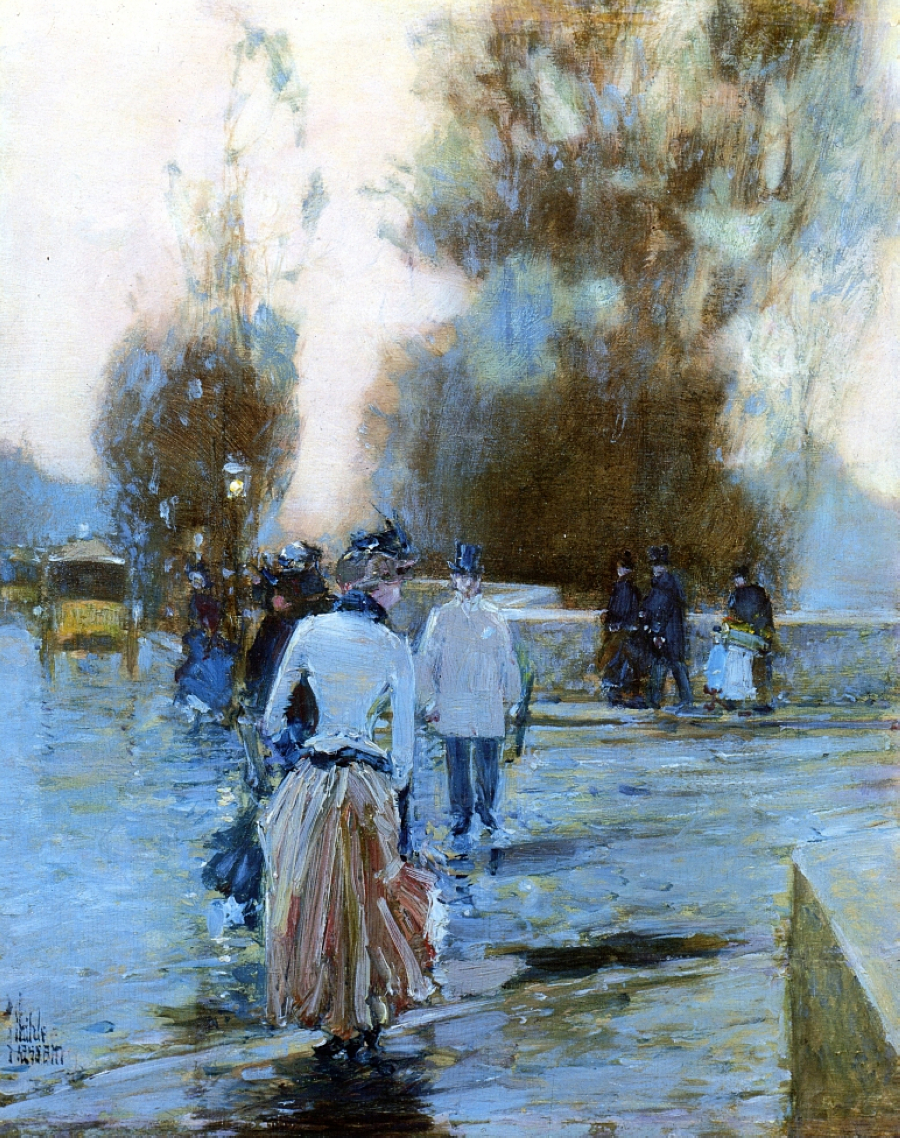This painting depicts a rainy city street scene with an impressionistic touch, highlighted by brush strokes and a washed-out color palette. Starting at the top left, the painting features areas of solid white, perhaps representing the sky or the diffused light of a rainy day. 

In the foreground, a woman in a white top with blue fringe and a pinkish-brown flowing skirt is walking away from us, her hat a soft blue. She appears to be holding a blue object in her left hand. To her right, a man in a white jacket and blue pants faces her, perhaps holding something in his left hand as well. The ground beneath them reflects light, creating a light blue sheen typical of wet surfaces.

To the left in the middle ground, a yellow vehicle resembling a taxi or a horse-drawn carriage stands out amidst the scene. Various figures in dark clothing, some carrying umbrellas, are dispersed throughout the background. On the far right, a group of three adults in dark clothing and two children in lighter attire walk alongside a short, brown-tinted wall that curves into the depth of the painting.

The background features two large, brown, tree-like shapes that appear dense at the base and become more diffuse as they rise, adding to the painting's dreamy, slightly unfocused atmosphere. Overall, the scene captures a timeless, rainy moment in a city, blending human activity with the elements.